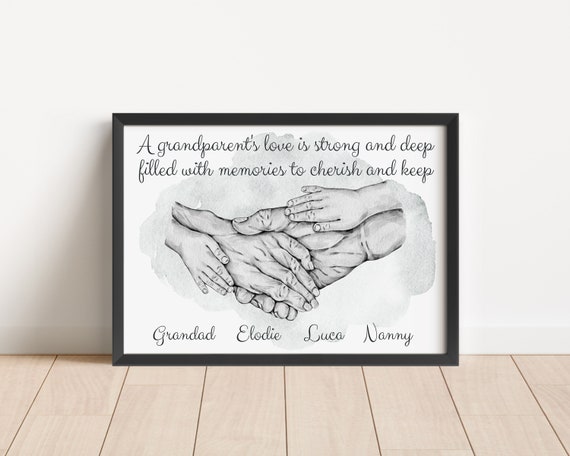This detailed photograph captures a touching black-and-white illustration framed in black and leaning against a plain white wall. The frame rests on a light tan wooden floor. The image, depicting a generational bond, features the hands of grandparents intertwined with those of their grandchildren. Specifically, it shows two larger hands—likely representing the grandparents—cradling two smaller hands, symbolizing the children's. Above this heartwarming scene, written in elegant cursive, is the phrase: "A grandparent's love is strong and deep, filled with memories to cherish and keep." Below the overlapping hands, the names "Granddad, Elodie, Luca, and Nanny" are inscribed, indicating the familial connection and love depicted in the drawing. This evocative picture emphasizes the strength and depth of a grandparent's love through the simple, yet profound, imagery of hands and the accompanying heartfelt text. The well-lit room highlights the sentimental value of the artwork and the cherished memories it represents.